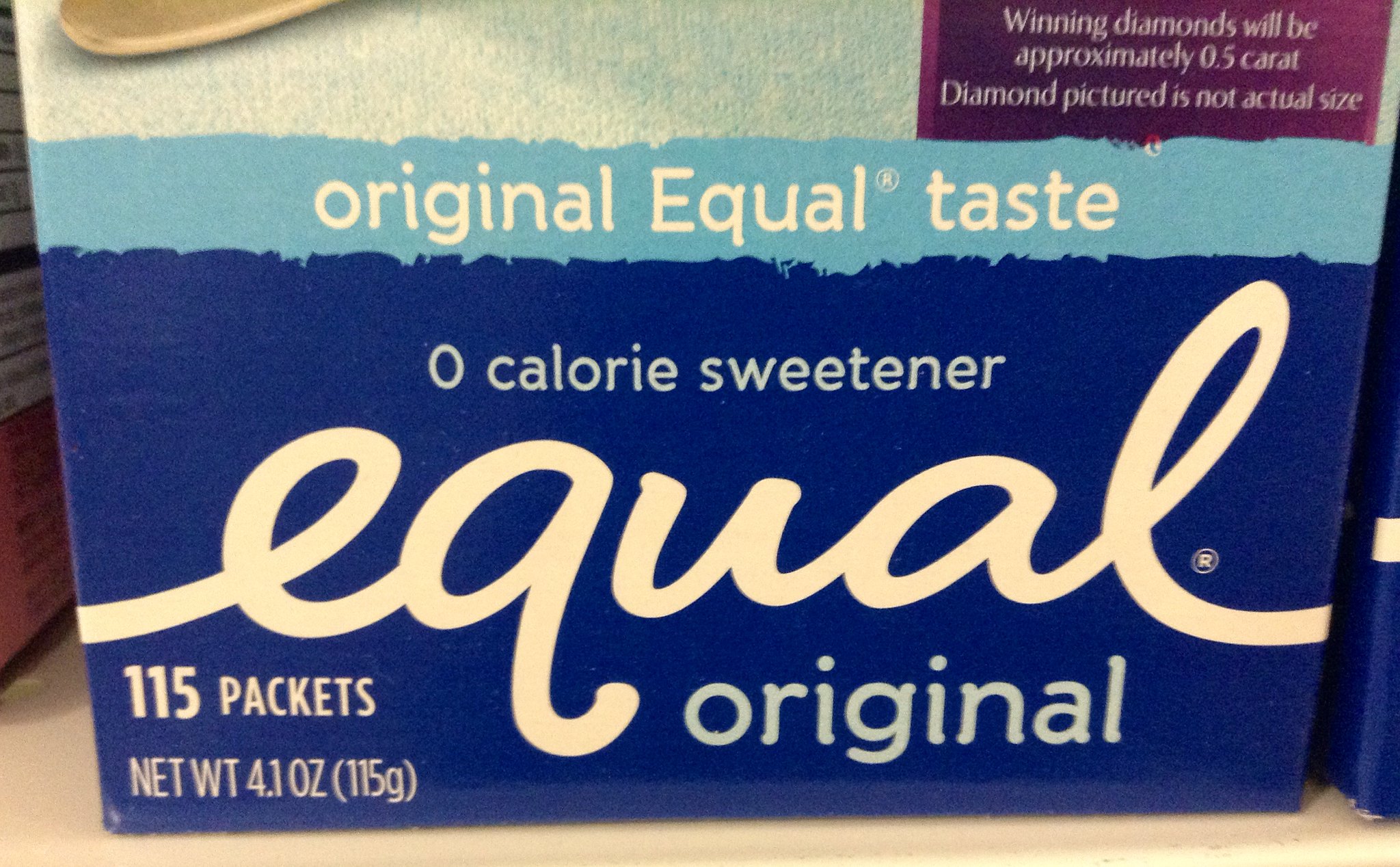This close-up photograph showcases a box of zero-calorie sweetener. The box features a light blue color at the top and transitions to a purple section in the upper right corner that bears the text: "Winning Diamonds will be approximately 0.05 carat. Diamond pictured is not actual size." Just below this area, there is a small tear, adding an element of imperfection to the packaging. Below the tear, the branding elements are visible, including the words "Original," "Equal," and a circled "R" trademark symbol, followed by the word "Taste." Further down, it states "Zero-Calorie Sweetener" in bold letters. The brand name "Equal" is prominently displayed in italicized script with a distinctive lowercase "e." Beneath the "e," the label specifies "115 packets, net weight 4.1 OZ" with the metric equivalent "(115G)" in parentheses. Directly under the letters "UAL" in "Equal," the word "Original" is printed once more, reinforcing the product's flavor variant.